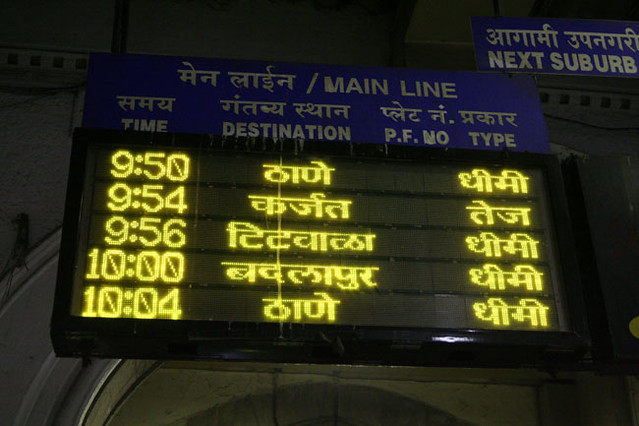The photograph captures a digital electronic display panel at a train station likely situated in the Middle East, suggested by prevalent Arabic text and architectural cues. The display panel prominently features a timetable, illuminated with yellow digital numbers showcasing departure times of 9:50, 9:54, 9:56, 10:00, and 10:04. Adjacent to these times are destination details written in white script on a blue background, presented in both Arabic and English. Adding to the multilingual nature, some text appears to be in other Asian scripts. Above the digital display, the upper portion features a sign with a light blue background, containing the phrase "NEXT SUBURB" in capital letters in English, preceded by text in a foreign script. This sign is positioned toward the upper right section of the image. The overall ambiance suggests it is nighttime, as inferred from the darkness outside, adding to the mystique and functionality of this transport hub's electronic guidance system.